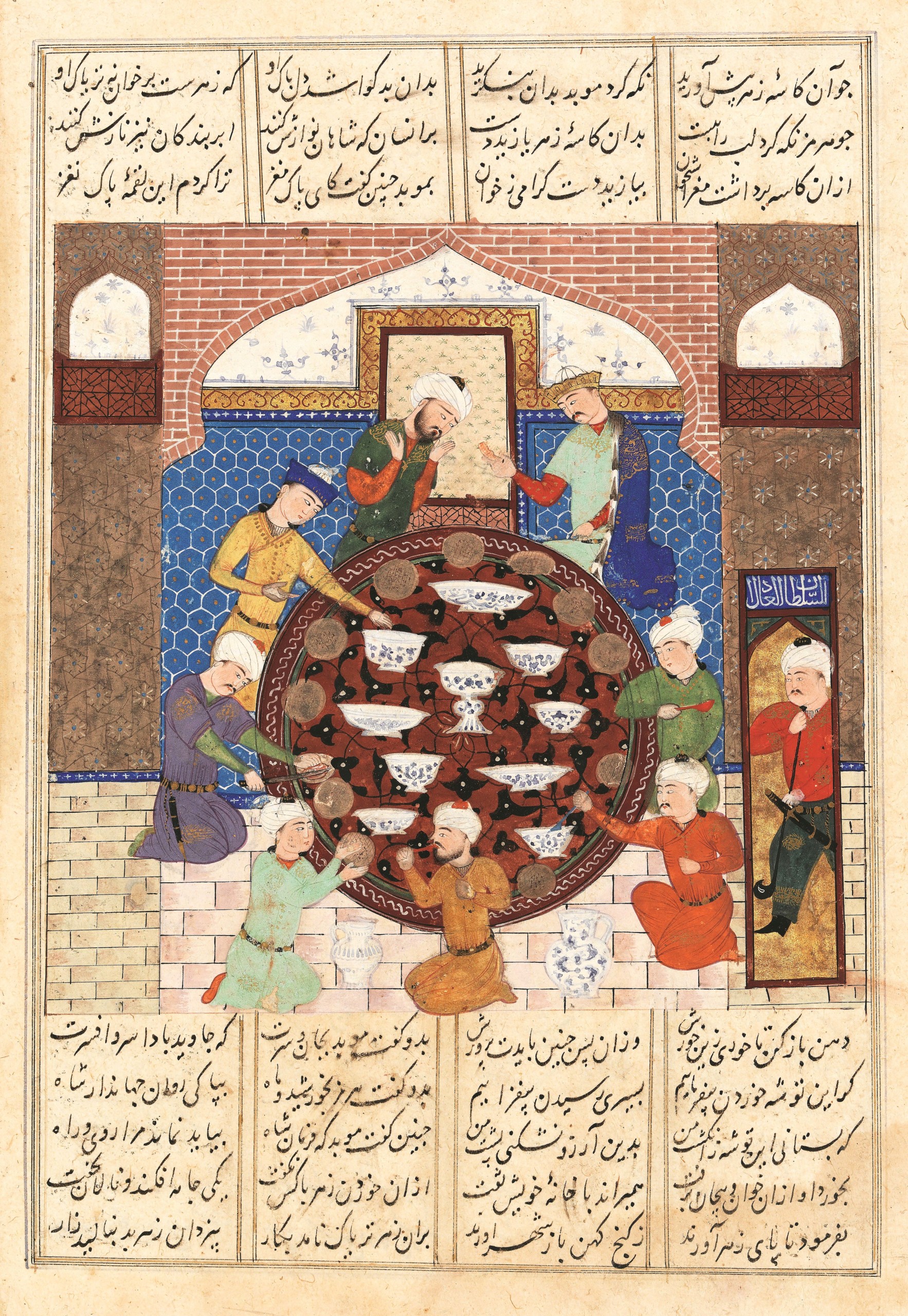The image, resembling a well-preserved page from an ancient manuscript, is bordered by a light brown parchment frame and features both artistic and textual elements. Measuring approximately five inches high and three to four inches wide, it houses a central illustration surrounded by blocks of Arabic script—four square blocks at the top and four vertical rectangles at the bottom. The text, rendered in a non-Roman script with elegant swoops and dots, adds a layer of historical context to the scene.

At the heart of the illustration is a circular, dark brown table adorned with an intricate black design. Around this table sit several men wearing white turbans and colorful robes in shades of brown, green, red, and yellow. Some men are engaged in conversation, others are reaching for white bowls and brown plates that are scattered around the table, indicative of a communal feast or significant event. Notably, one man is equipped with a sword at his hip, adding a sense of vigilance to the gathering.

The setting suggests an indoor environment, perhaps a temple, characterized by visible arches and a doorway or mirror on the right-hand side of the image. The detailed portrayal captures a moment of social and cultural interaction, framed elegantly by the surrounding Arabic script.